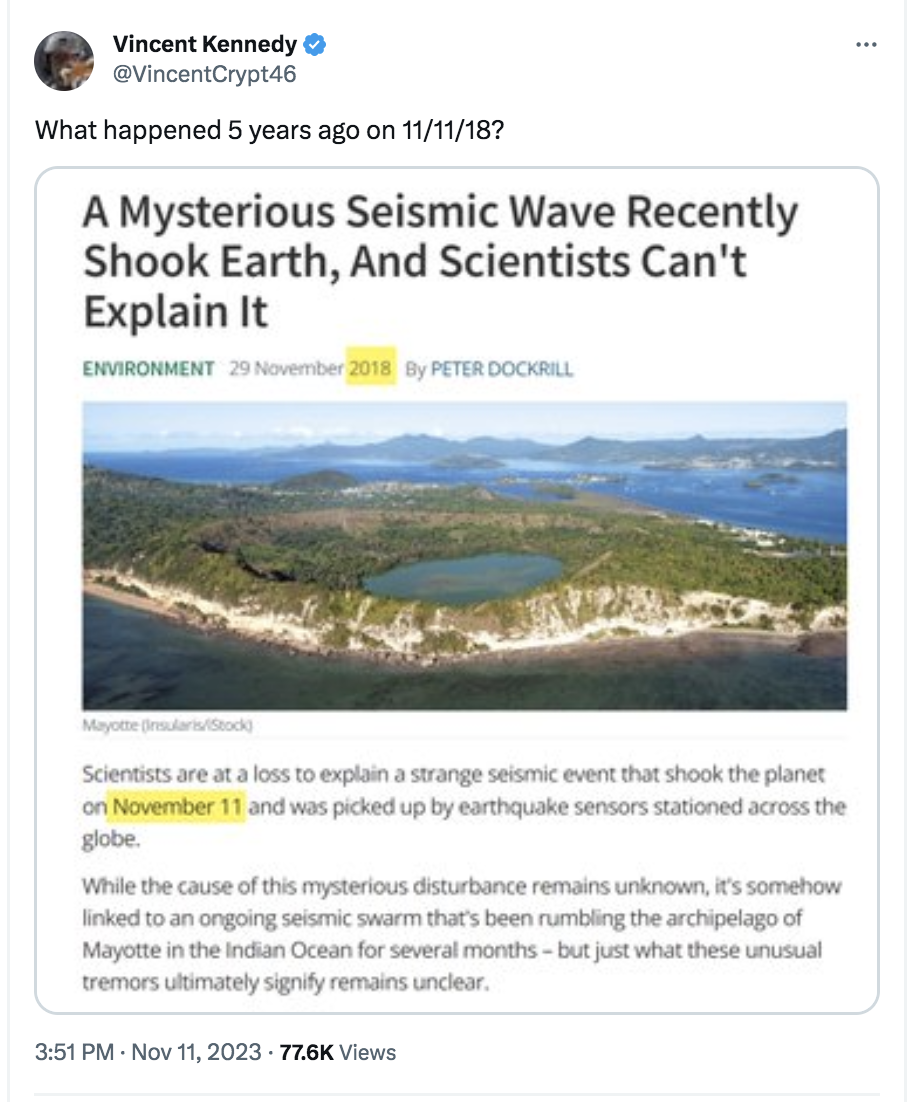A vertical screenshot from a social media platform, likely Twitter, posted by "Vincent Kennedy" (@VincentCrypt46), featuring a white background typical of a computer or smart device screen. The tweet includes Vincent's profile picture, a blue check mark indicating verification, and three horizontal dots on the right for additional options. The tweet, dated 11-11-18, asks, "What happened five years ago on 11-11-18?" Below this query, an article with a rounded box format is displayed with the headline, "A mysterious seismic wave recently shook Earth, and scientists can't explain it," written by Peter Dockrell in the environment section dated 29 November 2018. The article includes an image of calm waters and lush trees. The text explains that on November 11th, a mysterious seismic event was detected globally, linked to a seismic swarm in the Miao archipelago in the Indian Ocean. Despite the detection, scientists remain perplexed about the cause and significance of these unusual tremors. The tweet also displays the article's view count, date, and time of posting.